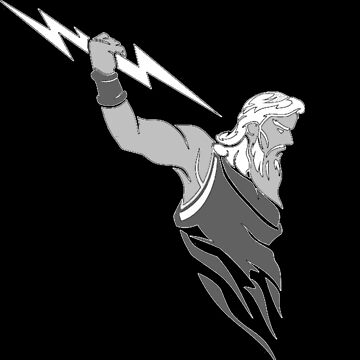In this black and white image, we see a detailed artistic depiction of Thor, the Norse god of thunder, holding a thunderbolt in his right hand. Thor is portrayed with flowing white hair and a big, long beard, both indicative of his venerable age and divine wisdom. His facial expression is one of intense anger, mouth open as if he's shouting, eyebrows furrowed to enhance his menacing glare. He wears a brown toga with a strap over his right shoulder, paired with a wristband or wrist guard on the same arm, further emphasizing his readiness for battle. His nose is prominently pointy, adding to his fierce demeanor. The lightning bolt in his hand is poised to be hurled, capturing a moment of divine wrath and impending action.